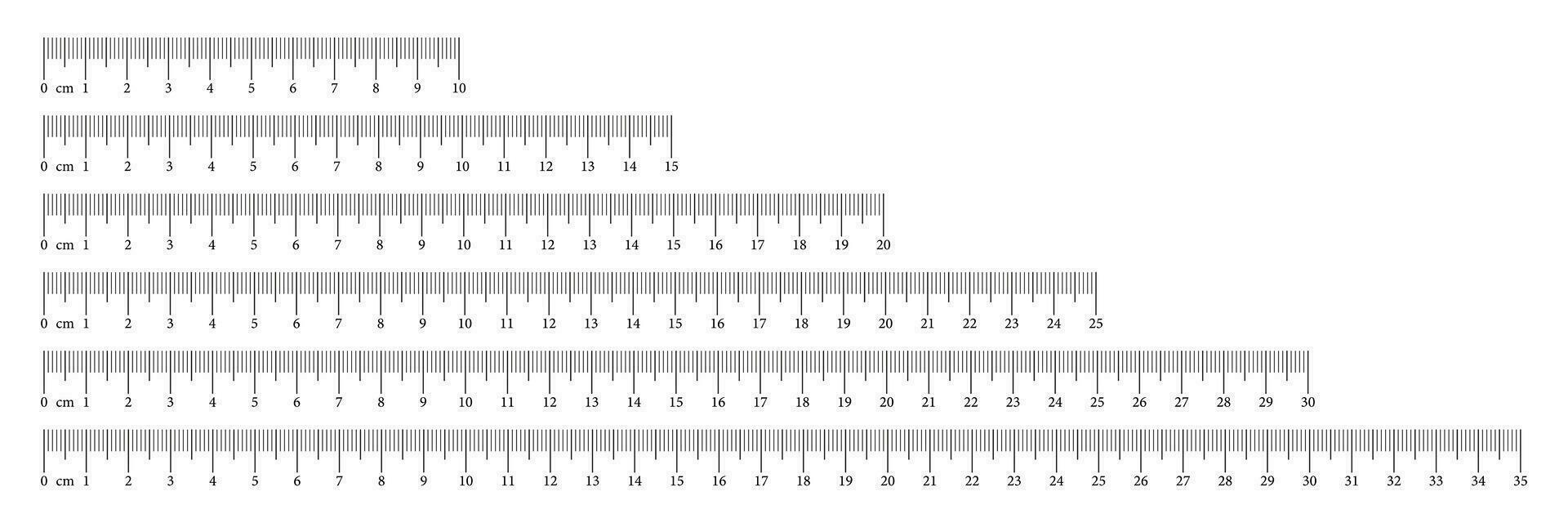The image features six rulers displayed in a descending staircase pattern against a plain white background. Each ruler is marked in black with clear, concise centimeter measurements starting from zero. The rulers increase in length from top to bottom: the top ruler extends to 10 centimeters; the second to 15 centimeters; the third to 20 centimeters; the fourth to 25 centimeters; the fifth to 30 centimeters; and the bottom one reaches 35 centimeters. The rulers only have whole number increments clearly marked, with a label indicating "centimeters" at the zero mark on the left side of each ruler.